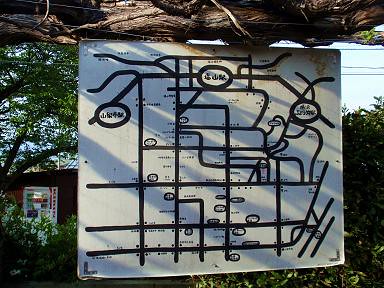The image features a white, square canvas or banner that appears to be somewhat weathered, with rust visible at the top right corner. The banner is hanging from what looks like a wooden tree branch, supported by a suspension wire beneath it. It is adorned with a network of connected black lines, both straight and curved, giving the impression of a complex, perhaps map-like design, possibly representing a park or theme park. In addition to the intricate lines, there are three prominent circles situated on the left, right, and at the top of the canvas. The background reveals a mixture of natural and man-made elements: a brown and light tan house with a glass-paneled white door is visible on the left, while power lines stretch overhead. The setting appears lush with trees, bushes, and additional signage visible further in the distance, suggesting a park-like environment.